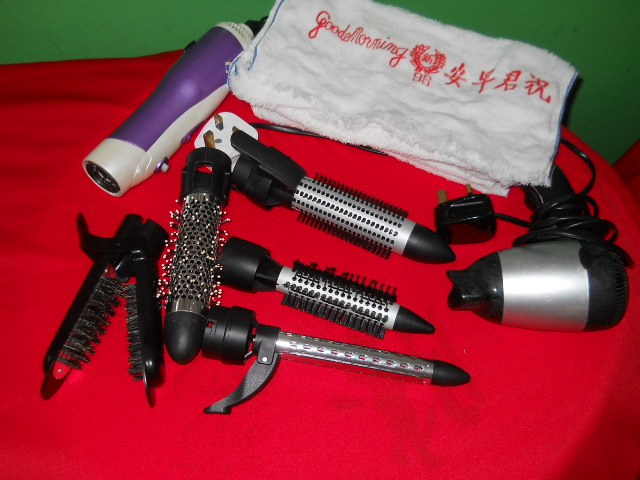This photograph captures an assortment of hair styling tools laid out on a table draped with a bright red cloth. Central to the image are various hairdryer attachments, including black and silver metallic pieces with bristles, elongated brushes, and a claw-like device that opens. To the right, there's a small hairdryer with its electrical cord neatly wrapped around the handle, while to the left, you see a white and red hair product with a long attachment. A folded white towel in the top right corner features text that says "Good Morning" along with Chinese symbols, all written in red ink. The background consists of a dark green wall, adding contrast to the vibrant red cloth below.